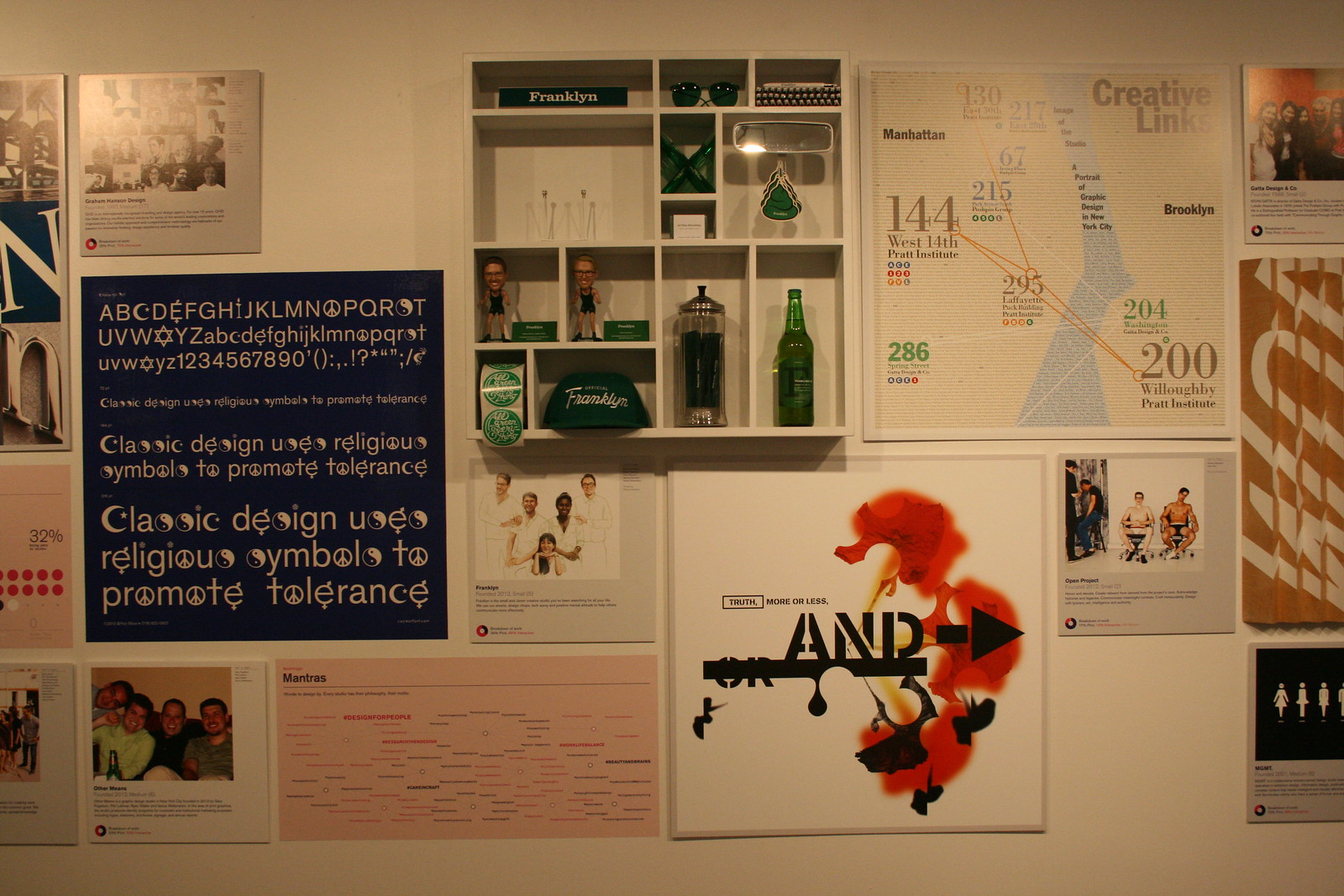This photograph captures a detailed and eclectic display typical of an art museum or gallery. A striking feature is a shelving unit on a white wall, adorned with various items such as a Heineken bottle, a coffee press, sunglasses with green lenses, air fresheners, a hat, and knickknacks, all arranged neatly. The wall is decorated with an array of posters and artworks, showcasing diverse content and styles.

To the left of the shelving unit, there is a large blue poster featuring an alphabet where several letters are substituted with religious and cultural symbols, such as a peace sign for "O," a yin-yang for "S," and the Star of David for "X." The text on this poster states, "Classic design uses religious symbol to promote tolerance," repeating and enlarging three times. Other posters exhibit a variety of themes and colors, including dark and white artwork, black and orange accents, and some blue elements.

A photograph on the top left displays a collage of people with very small text, while below it, another image portrays friendly individuals. Adjacent is a pink flowchart poster, likely depicting a series of connections. Above the shelving unit is a white picture with multicultural figures. Further to the right, there is a creative links poster, presenting a map of Manhattan with various numbered points of interest.

This curated arrangement creates a vibrant and visually stimulating environment, blending physical objects, print media, photography, and graphic design, emphasizing themes of multiculturalism and tolerance within an artistic setting.